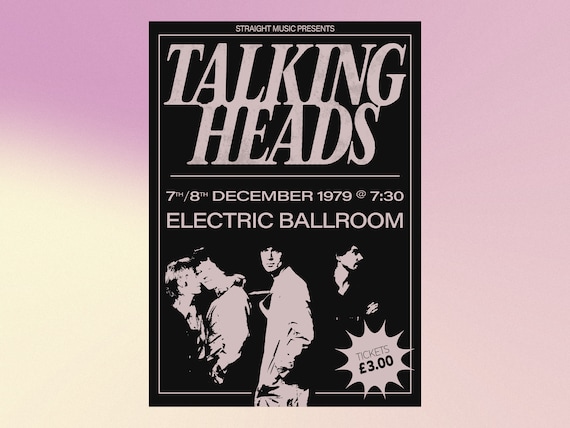The poster promoting the band Talking Heads features a striking black background with an ombre effect of pink, cream, and yellow. The top of the poster reads "Straight Music Presents" in pinkish-hued text. Below, the band's name, "Talking Heads," appears prominently in a similar color. The dates "7th-8th December 1979" and the venue "7:30 Electric Ballroom" are listed underneath the band's name. The poster also displays black-and-white images of the band members positioned in the middle – one in the center, another to the left with a lady, and a third on the right, potentially in a sewer-like setting. In the bottom right corner, the ticket price is noted as £3, indicating the event's British location. The overall design is accented by a thin white stripe running about a quarter inch inside from the edges.